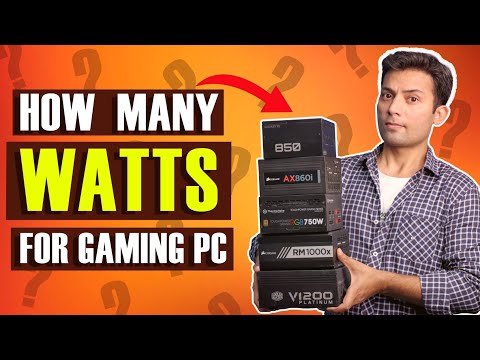A computerized image designed as a YouTube video thumbnail features a young man, aged about 25 to 30, holding five old gaming PC component boxes. The caption above and below the main image reads, "How many watts for gaming PC?" in white and yellow text, accompanied by a red arrow pointing to the boxes. The background is a vivid orange with scattered question marks, hinting at an educational theme. The young man, who has neatly combed short brown hair and is clean-shaven, stands on the right side of the image. He wears a blue and white small checkered shirt with rolled-up sleeves over a white undershirt. He gazes directly into the camera without smiling. The boxes he holds are labeled with different power ratings: V12 Platinum, RM1000X, 750W, AX860i, and AX850.